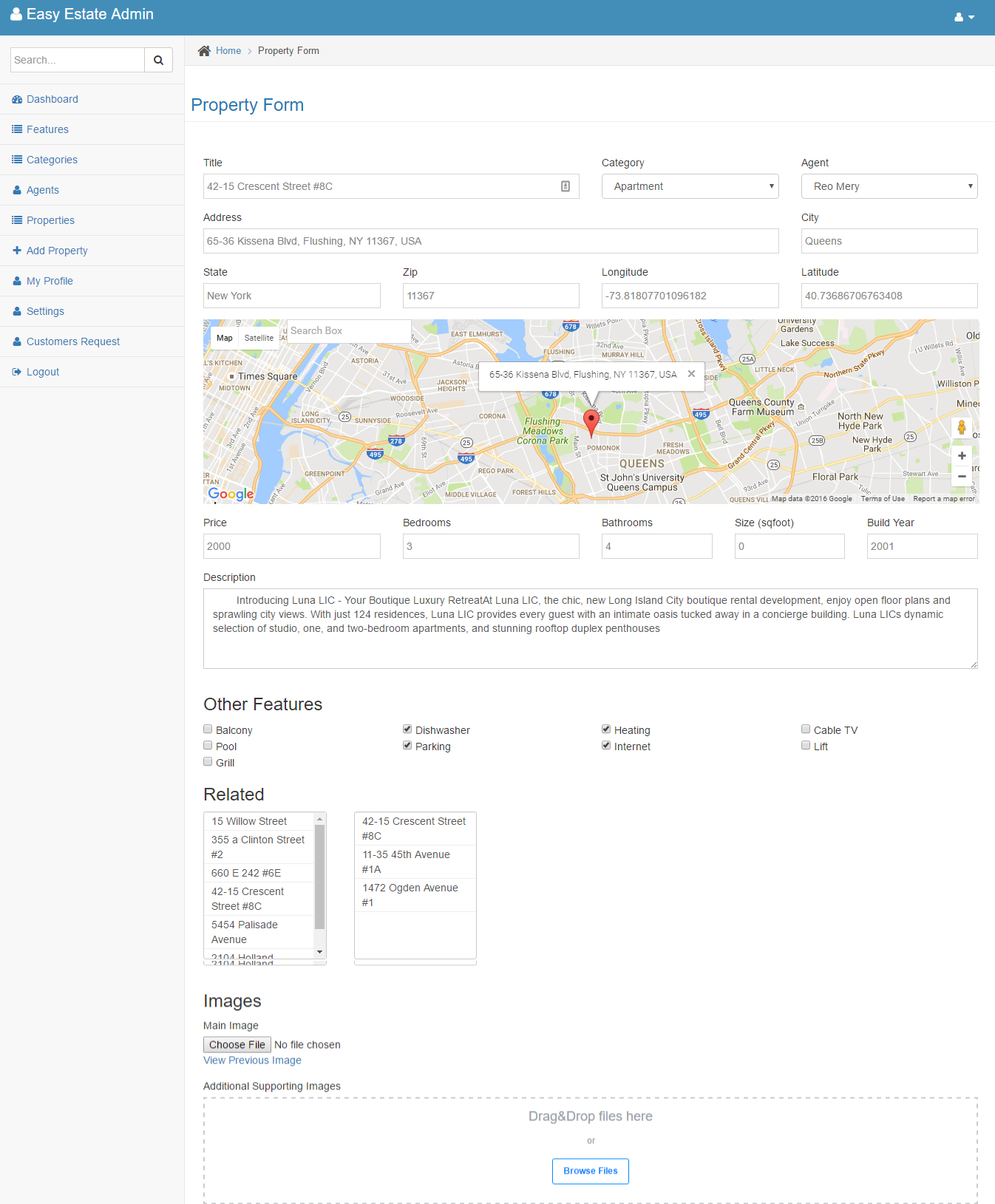The image depicts a website interface for "Easy Estate Admin" with a light blue banner at the top. The banner features the text "Easy Estate Admin" in white on the left side and includes a white human profile icon with a down arrow for login options on the right. 

On the left side of the image, there's a sidebar with a search bar at the top, followed by a menu with blue text items against a light gray background. The menu items are: Dashboard, Features, Categories, Agents, Properties, Add Property, My Profile, Settings, Customer Requests, and Logout.

Centered at the top of the image is a section with a white background displaying a form titled "Property Form" in blue text. The form includes fields such as Title, Category, Agent, Address, City, State, Zip, Longitude, and Latitude. Below these fields is an embedded Google Map with a red marker indicating the location based on the entered latitude and longitude.

Further down the form, there are more fields to input details like Price, Bedrooms, Bathrooms, Size, Optional Build Year, and a large rectangle for the property Description. Below this section, there is a checklist with options for various property features: Balcony, Pool, Grill, Dishwasher, Parking, Heating, Internet, Cable TV, and Lift.

At the bottom of the form, there are sections for Related Menu and Images. For images, there is an option to upload the main image with a "Choose File" button indicating "No file chosen," and additional supporting images can be uploaded via a drag-and-drop interface. The form is concluded with a blue button labeled "Browse Files" for file selection and uploading.